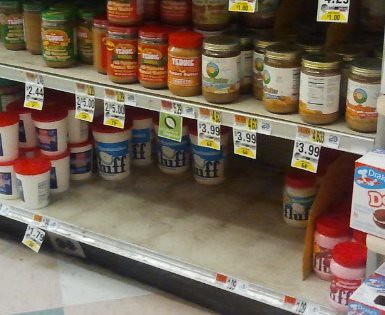This indoor color photograph, taken at a slight angle, captures two shelves in a grocery store with a portion of the linoleum tile floor visible in the lower left corner. The bottom shelf is sparsely stocked with about five to six white cylindrical containers, each with a red cap and blue lettering that reads "Fluff," likely referring to marshmallow cream. The shelf above is filled with various jars, some with red, silver, or gold caps. Although the labels are out of focus, the red-topped jars appear to contain peanut butter, while the others might hold canned or jarred fruits. Various price tags are visible along the edge of both shelves, displaying prices like $3.99 and offers such as two for $5, all in American dollars. The juxtaposition of the almost empty bottom shelf with the more densely packed upper shelf, along with the detailed price tags, offers a snapshot of the store's inventory and pricing.